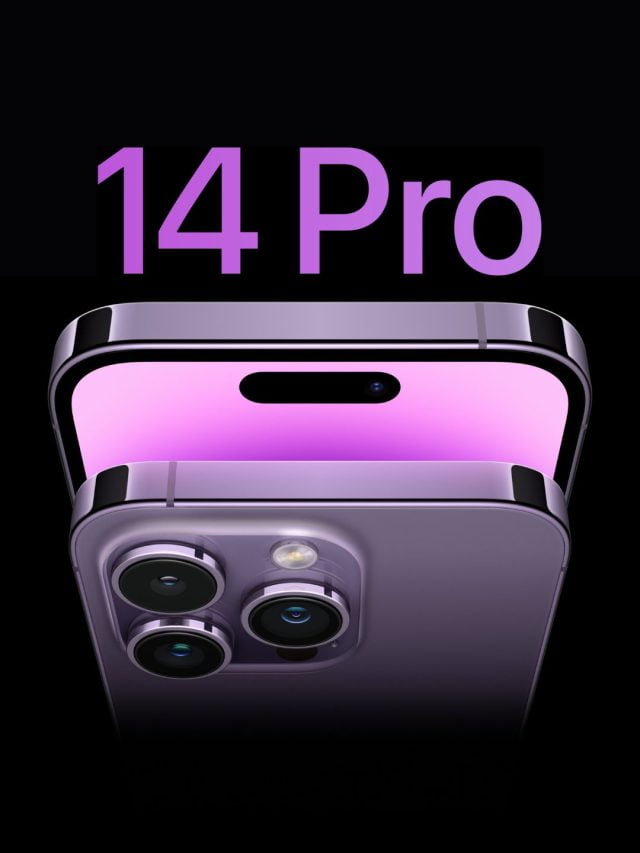The image showcases a product advertisement, specifically highlighting a cell phone prominently. Captured from a top-down perspective, the image focuses on both the front and back views of the device's upper half. The phone features a sleek design with dark gray sides and a light gray back. Displayed at the top of the advertisement, the text "14 Pro" is written in vibrant purple.

The phone's back reveals a sophisticated camera setup within a left-aligned square module. It comprises three lenses: two aligned vertically on the left and one centrally placed on the right. Adjacent to the lenses is a small, white circular element, identified as the flash, likely serving as both a flashlight and photo flash. 

On the front, a horizontal black oval sits centrally at the top, accompanied by a small blue square to its right, possibly indicating a sensor or additional camera feature. The advertisement is set against a completely black background, which accentuates the phone's details. The brand of the phone isn't mentioned, leaving the text "14 Pro" as the sole identifier of the model.